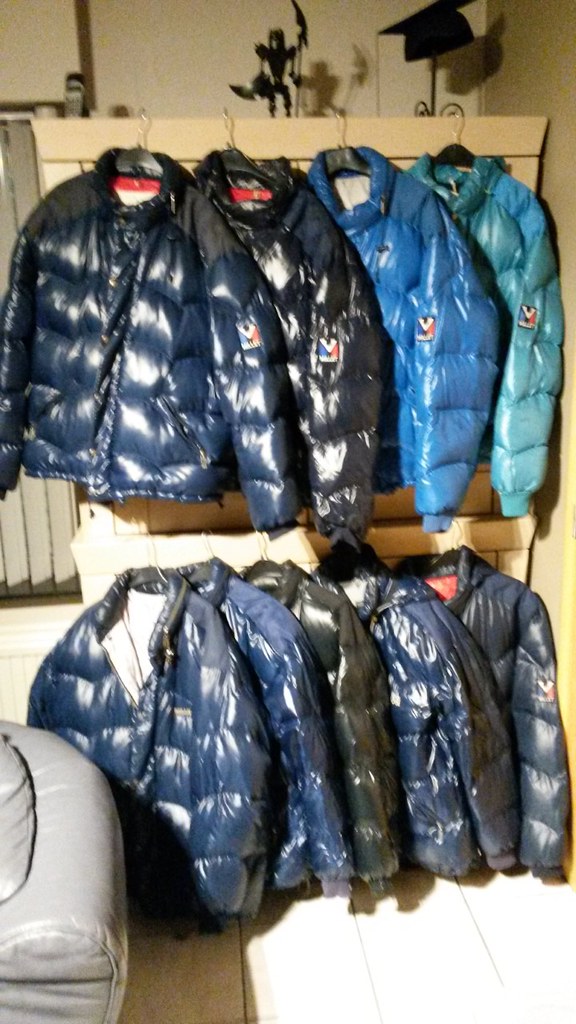The image depicts a brightly lit room featuring a collection of winter bubble jackets, neatly arranged on a shelving system with two tiers. On the upper tier, four puffer coats are hung: a teal blue jacket, a medium-tone blue jacket, a black jacket, and another shade of blue jacket, each with a reflective, water-repellent finish. The lower tier holds five more jackets: three in various shades of navy blue, one shimmering blue, and one black. Each jacket on the bottom tier hangs beneath the corresponding jacket above it. The jackets are organized with attention to detail, and one of the navy blue jackets on the lower tier is distinguished by a red inner collar. On the far left of the image, there is a gray leather couch, and on the top right, a black graduation hat is visible. The background includes vertical blinds in an off-white color and a brownish panel flanked by light brown walls, adding warmth to the room’s ambiance.